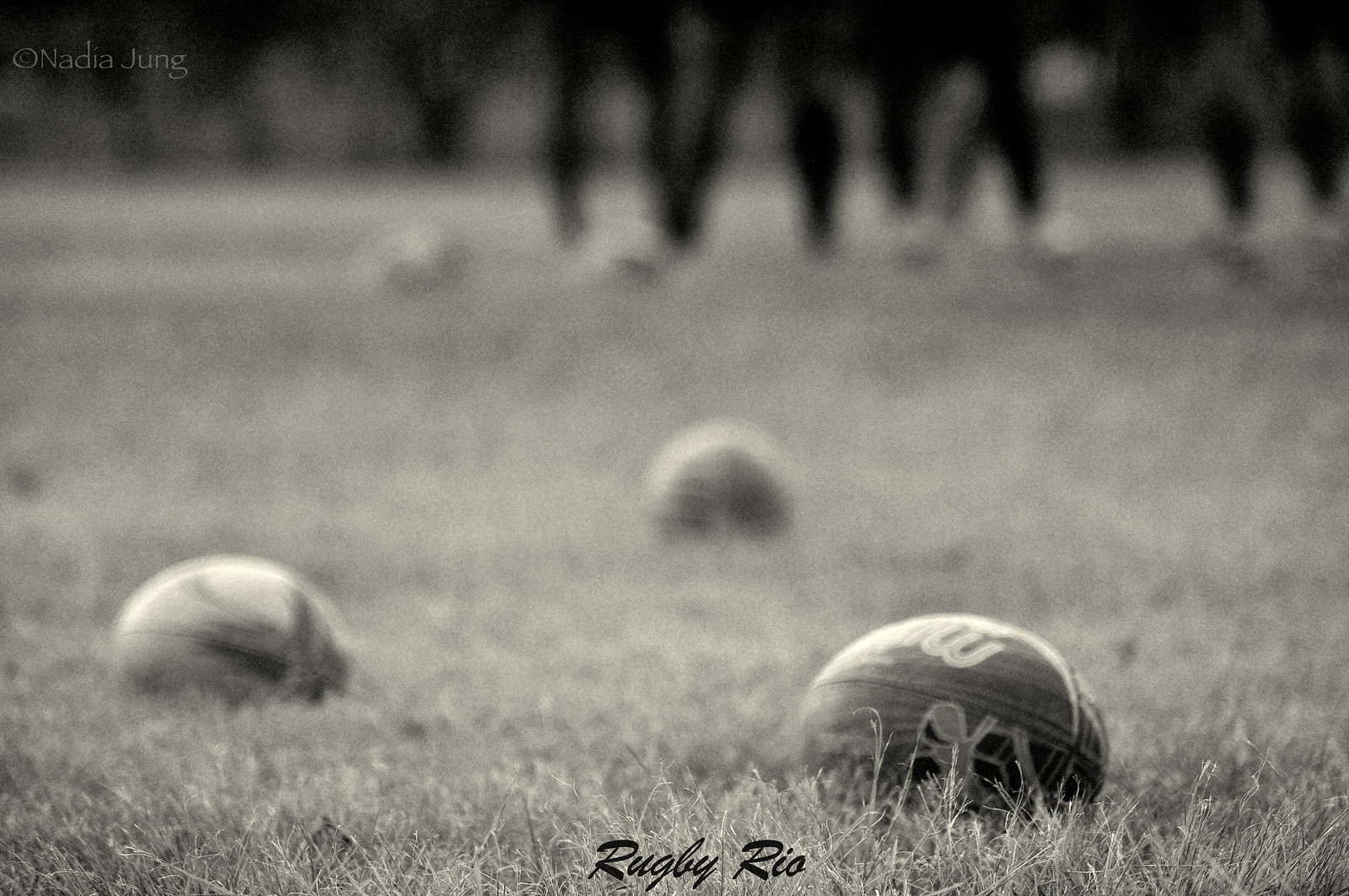In a black-and-white photograph, a grassy field, with grass approximately one inch high, extends across the foreground. Scattered on the grass are four rugby balls, the nearest one almost in focus and revealing a dark and light pattern. In the dark, blurry background, four figures stand at a distance, their legs and possibly black pants faintly visible. Overlaid text at the bottom of the image reads "Rugby Rio" in bold black print, hinting at an upcoming rugby game or practice. Additionally, in the top left corner, the name "Onada JUNG" is prominently displayed in capital letters. The entire image, devoid of color, exudes a grayscale ambiance with varying shades of black and gray.